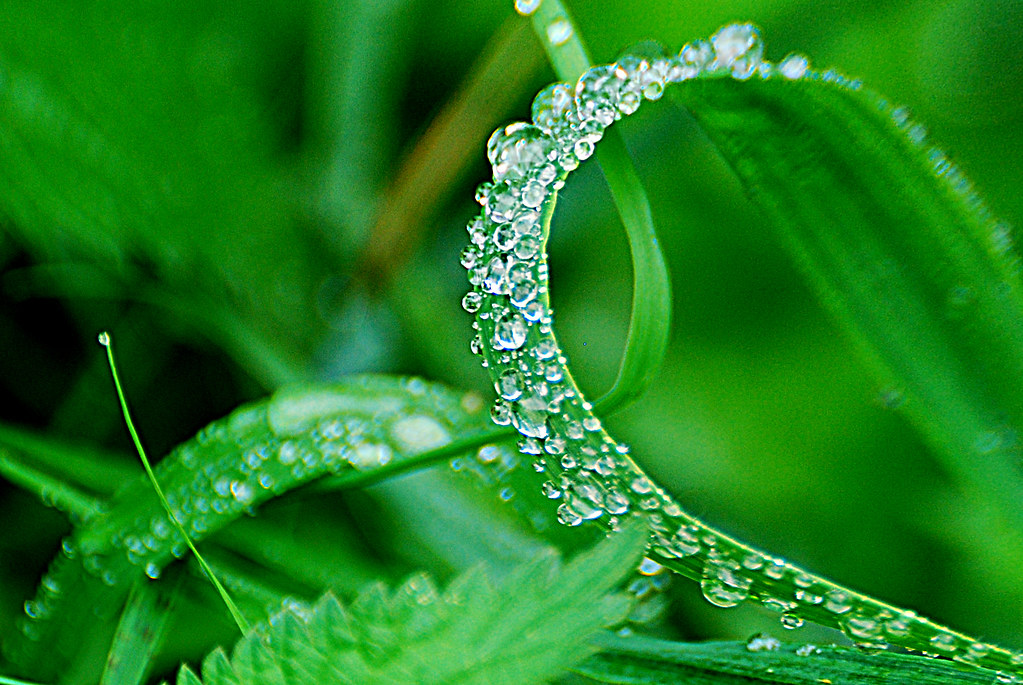A vivid close-up reveals a bright green, pointed leaf, curved almost into an oval, glistening with numerous clear, crystalline water droplets. The leaf's vibrant green surface is adorned with tiny beads of water, starting from its base and covering it entirely as it curls gracefully upward to the right. Surrounding this focal leaf are other leaves, also wet and varying in appearance; one appears open and similarly covered in dew, while another resembles a light green Christmas tree leaf with a tiny water droplet atop a long strand. The blurred green background enhances the sharp, detailed depiction of the leaves in the foreground, emphasizing the shallow depth of field and drawing the observer’s eye to the intricate, glistening water droplets.